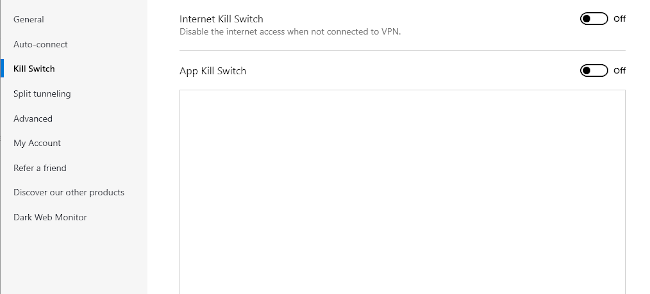A cropped screenshot of the VPN settings interface is displayed. On the left side, there is a grey vertical panel featuring a list of categories: General, Autoconnect, Killswitch (highlighted in bold black font with a vertical blue line beside it), Split Tunneling, Advanced, My Account, Refer a Friend, Discover Our Other Products, and Dark Web Monitor. The main section to the right of the panel has a white background. At the top left, the title "Internet Killswitch" is in black font, followed by the subtitle "Disable Internet Access When Not Connected to VPN" in bold grey letters. To the right of this subtitle is a toggle switch indicating the function is off. Further down, "App Killswitch" is labeled in smaller black letters, accompanied by another toggle switch on the far right, also set to off.